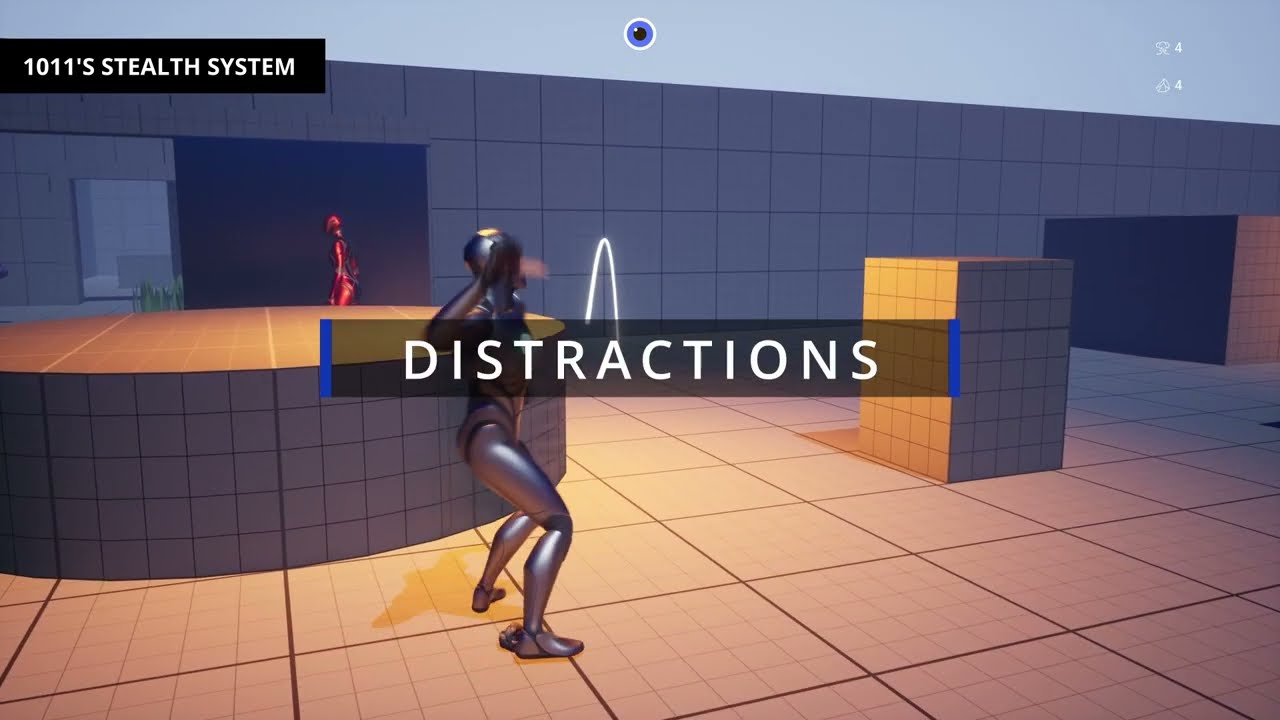The scene is set in what appears to be a digital drawing or screenshot from a video game or animated setting, featuring a silver robot-like figure standing outdoors in front of a gray tiled building. The floor also consists of the same gray tiles. Dominating the center of the image is the silver robot, clad in a skin-tight suit, with its right arm raised as if poised to throw something. A large, round pillar tiled similarly to the wall and ground stands adjacent to the robot on the left. Further in the background to the left is another character, a robot in red.

Several distinct elements define the scene's environment: a large square pillar close to the wall, brown in color, and another square pillar in the middle of the ground, depicted in a goldish yellow shade, both matching the general tiled aesthetic. Floating text overlays the scene: a transparent black rectangle centered both vertically and horizontally bears the word "DISTRACTIONS" in white lettering. In the upper left-hand corner of the image, white text over a black bar reads "1011S STEALTH SYSTEM," suggesting a possible security system interface. Additionally, the background reveals a dark grey square-paneled wall reaching up to a light blue ceiling, which features a central dark blue and gray circle outlined in white, possibly indicating a security camera. To the right of the scene, a column tiled in light tan and brown catches the robot’s attention, with an apparent opening in the wall behind the column, implying a potential passageway.